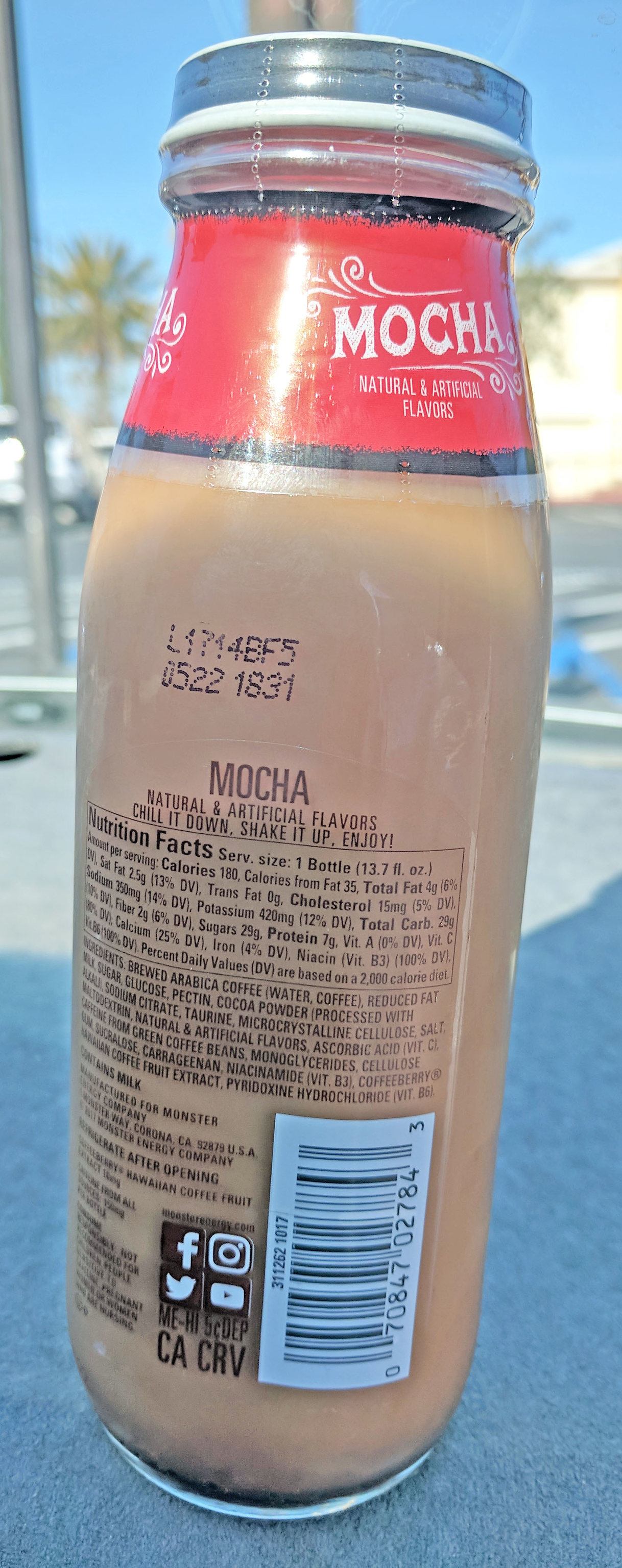This is a detailed color photograph capturing a tall, slender glass bottle of mocha-flavored iced coffee, sealed with a black screw-on lid accented with a white border and additional shrink-wrap around the cap. The bottle prominently features a bold red label that circles the entire bottle, displaying the words "mocha with natural and artificial flavors." Positioned below the lid, the label includes nutritional facts, ingredients, and a series of inventory numbers such as L171FB5, 0522-1831. Additional label details read, "Chill it down, shake it up, enjoy," and "Contains milk, manufactured for Munster." Social media icons for Facebook, Instagram, Twitter, and YouTube are visible, along with a black and white vertically aligned barcode, and text that mentions ME-HI 5 cent deposit and California CRV. The bottle is set against a vibrant backdrop featuring a bright blue sky, large palm trees, and a visible parking lot with some cars. The surface it rests on appears to be gray cement, reinforcing the on-the-go convenience store feel of the scene.